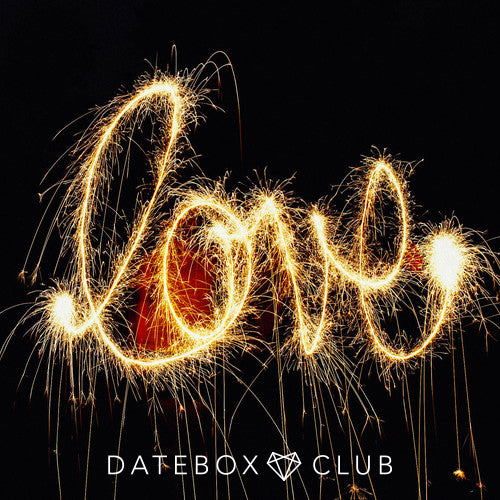The image features a nighttime scene with a dark, black background reminiscent of the night sky. At the bottom of the image, in white text, it reads "Datebox Club," with a diamond-shaped heart symbol between the words "Datebox" and "Club." Dominating the center of the image, the word "love" is elegantly written in a cursive script using sparklers. The sparklers create bright yellow and orange, fiery trails that spell out the word, giving a vivid, sparkling effect. Behind the word "love," there is a faintly visible subject, possibly the person creating the sparkler script, who appears to be wearing a red jacket. The intricate details of the sparkler trails against the dark backdrop create an enchanting and festive atmosphere.